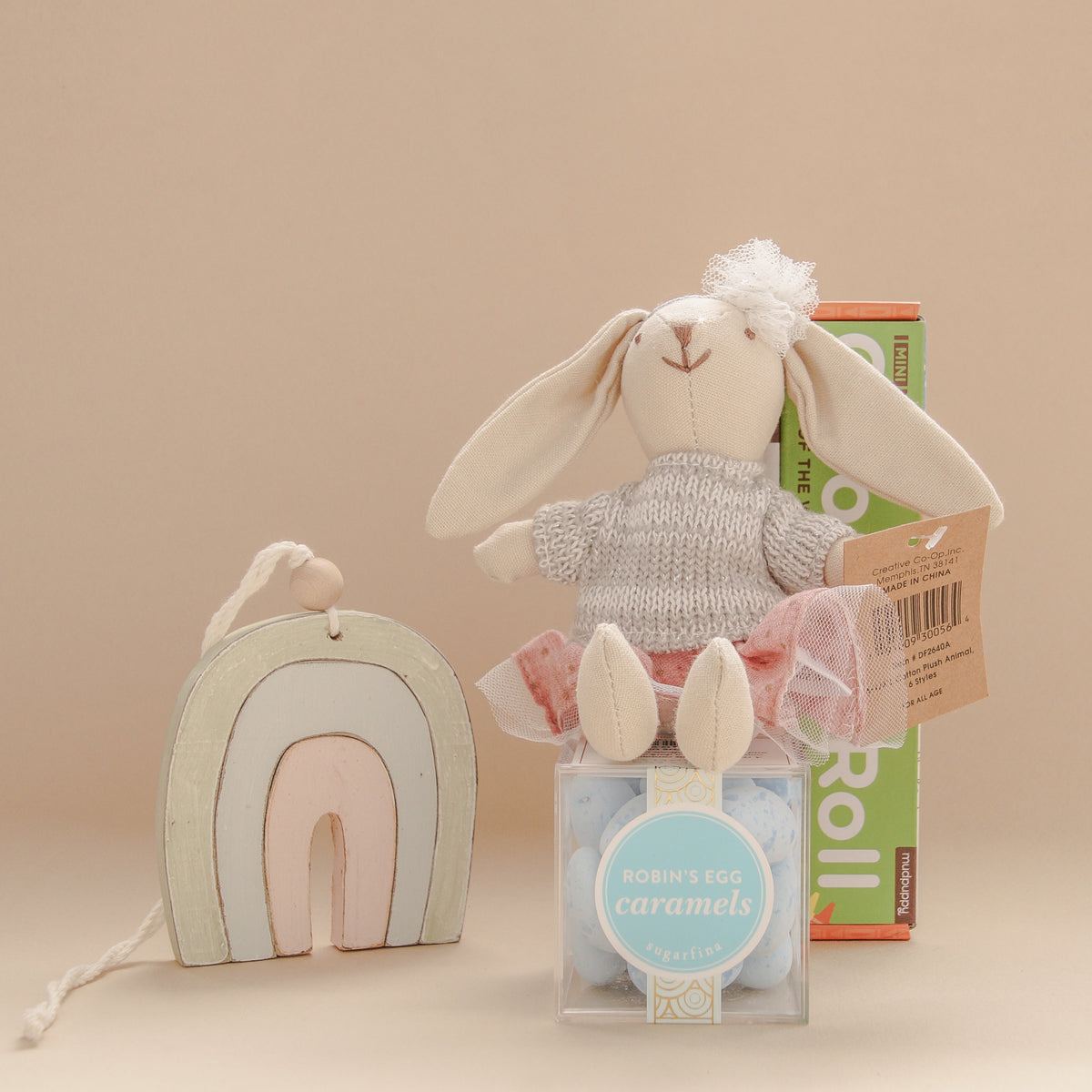The image is a detailed scene featuring a pink background. Central to the image is a soft bunny toy, dressed in a sweater, pink skirt, and a white headband, seated atop a rectangular plastic box. The box displays the label "Robin's Egg Caramels" and contains blue objects inside. Nearby, on the left side, appears a horseshoe-shaped item consisting of three layers: an outer green layer, a central blue layer, and an innermost pink layer, with a thread attached to its top. Behind the bunny, a green box is partially visible, with some identifiable text including “Creative Co-op Inc,” along with a barcode and other descriptive phrases. Additionally, there is a small rainbow adjacent to the bunny, adding a whimsical touch to the scene. This carefully arranged display could be interpreted as part of a baby product set or a gift hamper.